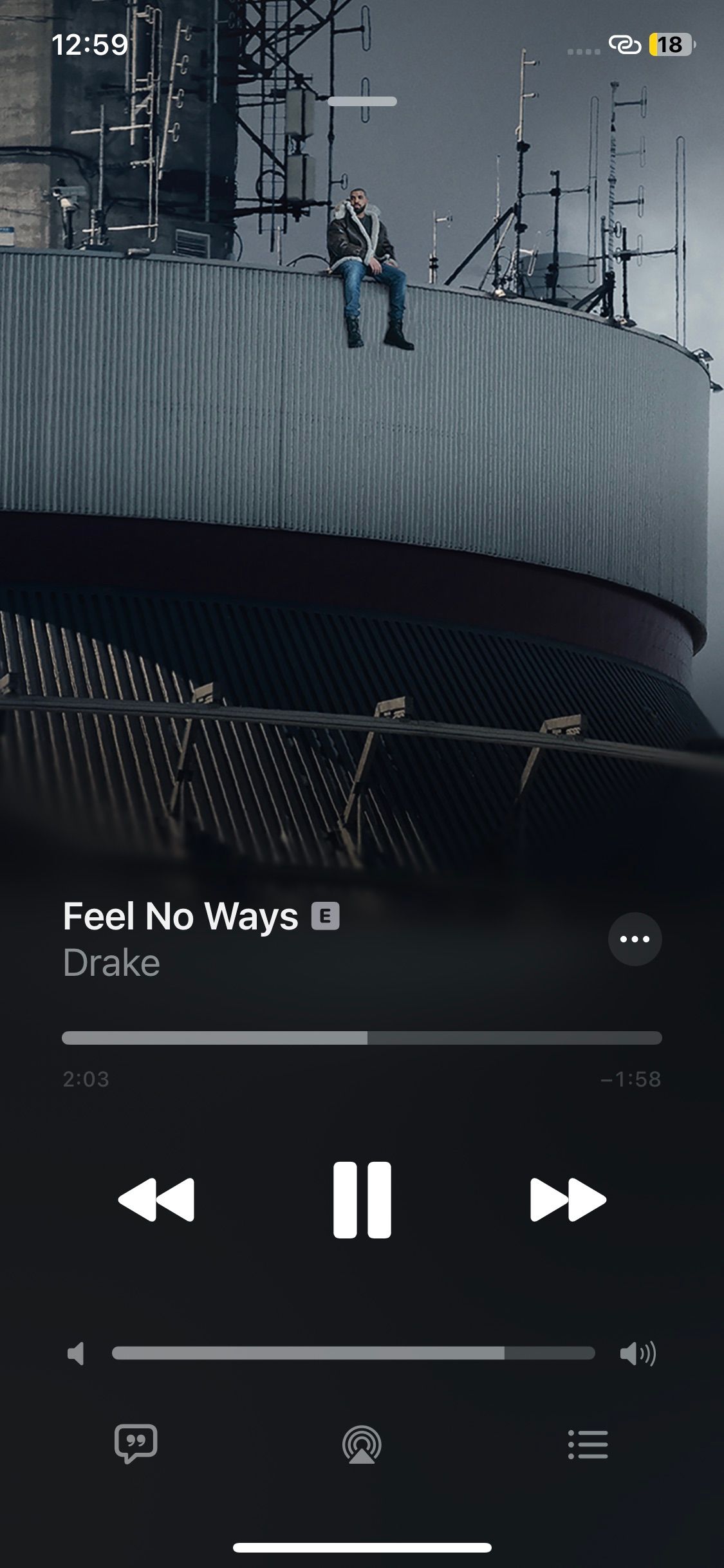This screenshot captures the interface of a music streaming app featuring a track by Drake, titled "Feel No Ways." The image displayed within the app is of Drake sitting alone on the edge of what appears to be a ship's ledge, exuding a contemplative vibe. He is dressed in a stylish black leather coat lined with white Sherpa, paired with dark blue jeans and black military-style combat boots. The playback of the song indicates that it is two minutes and three seconds into the track with a remaining duration of one minute and 58 seconds. 

Visible on the interface are the rewind, pause, and fast-forward buttons. The volume is set quite high, as depicted by the volume bar almost reaching its maximum level. Additional icons at the bottom of the interface include a message button, a share button, and a menu button. At the top, typical status indicators are visible, showing the current time as 12:59 and a low battery level of 18%.